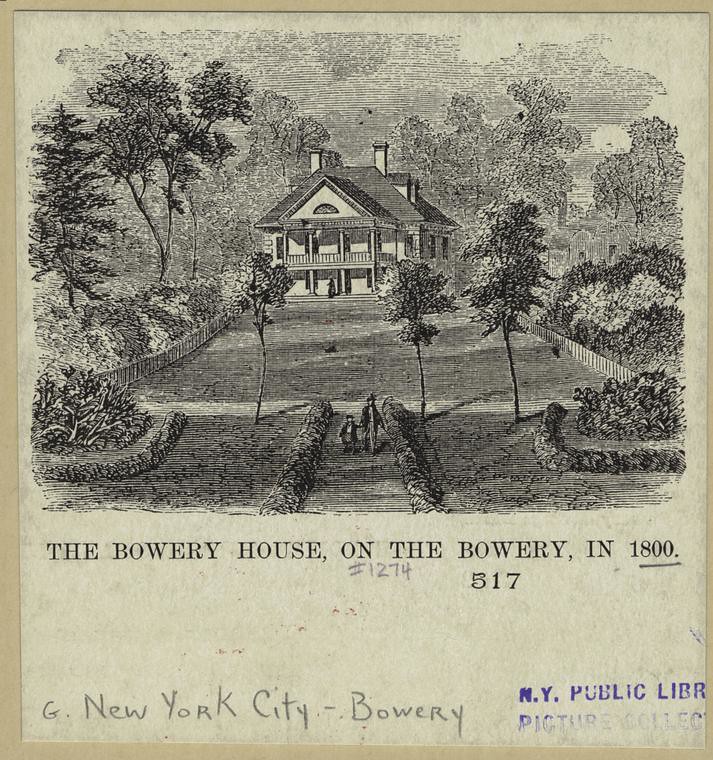The image is a scanned illustration resembling a historic card placed in a book. It features a detailed pencil drawing that occupies the top two-thirds of the page, showcasing a grand two-story house with an attic and multiple chimneys. The house is fronted by columns and surrounded by a sprawling landscape with trees and hedgerows. A large driveway runs from left to right, intersected by a pathway leading directly to the house. Along this pathway, two human figures—a shorter person holding hands with a taller one—are depicted walking towards the house, while another figure stands on the porch. The borders of the page are tan, contrasting with the white background of the drawing. At the very bottom, the text reads: "The Bowery House on the Bowery, IN 1800-517," with an additional pencil notation on the bottom left stating, "G. New York City, Bowery."